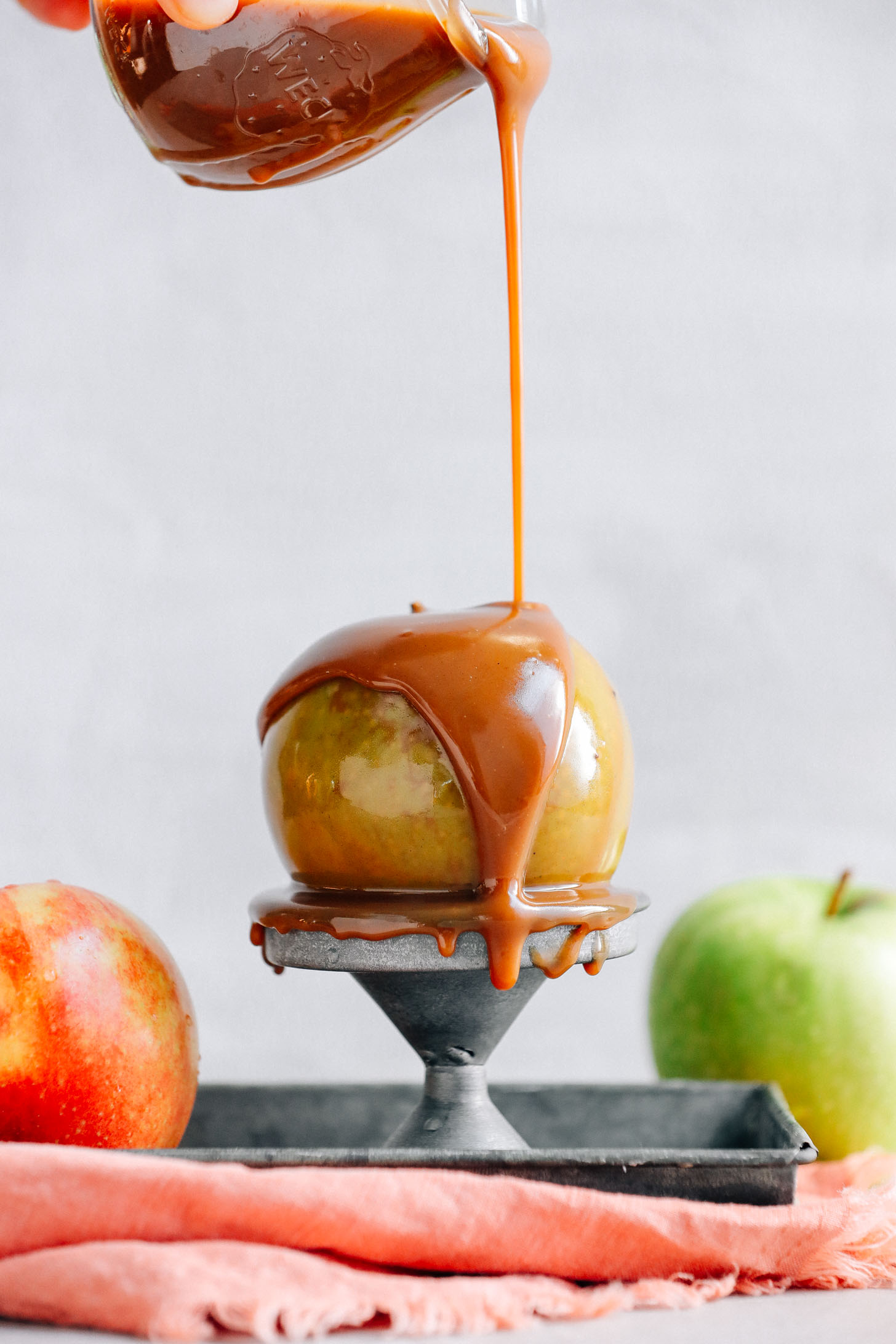In this elegantly composed image, we witness the intricate process of making a caramel apple. Central to the scene is a shiny green apple placed on a rustic metal pedestal, set within a rectangular sheet pan to catch the luscious caramel drips. Above, a hand obscured partially from view carefully pours thick, glossy caramel from a glass jar labeled "Weck," creating a mesmerizing stream that cascades over the apple, enveloping it in sweet, molten caramel. 

Out of focus, a red apple rests within the sheet pan to the left of the pedestal, while another green apple sits in the background, blending softly into the image's greyish, hazy backdrop. A peach-hued towel peeks from underneath the pan, adding a touch of warmth to the overall composition. The tightly focused depth of field highlights the rich texture and irresistible appeal of the caramel-covered apple, suggesting a scene straight out of a high-end food blog or a gourmet cookbook.